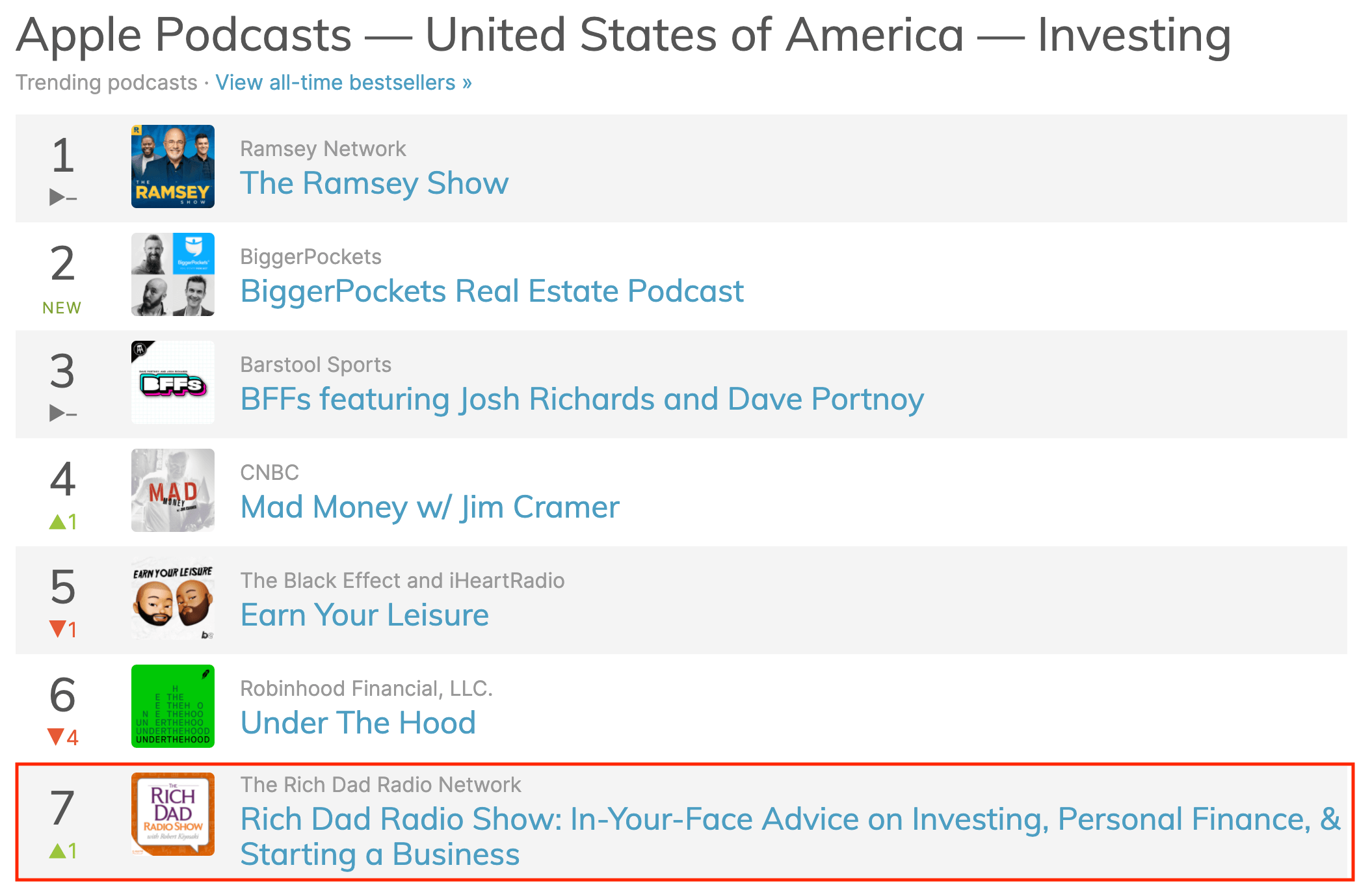This screenshot showcases a segment of a website featuring the top trending investment podcasts in the United States, as listed on Apple Podcasts. The header, in bold black font, reads "applepodcasts-unitedstatesofamerica-investing." Below this header is a clickable link labeled "trendingpodcastsviewalltimebestsellers."

The main content is a vertically arranged list, ranking podcasts from 1 through 7. Of particular note, the 7th position is highlighted with a red border, indicating its importance.

The rankings are as follows:
1. **The Ramsey Show** by Ramsey Network
2. **BiggerPockets Real Estate Podcast**
3. **BFFs featuring Josh Richards and Dave Portnoy** from Barstool Sports
4. **Mad Money with Jim Cramer** by CNBC
5. **Earn Your Leisure** by The Black Effect and iHeartRadio
6. **Under the Hood** by Robinhood Financial LLC
7. **Rich Dad Radio Show** by The Rich Dad Radio Network, highlighted with a red border and featuring in-your-face advice on investing.